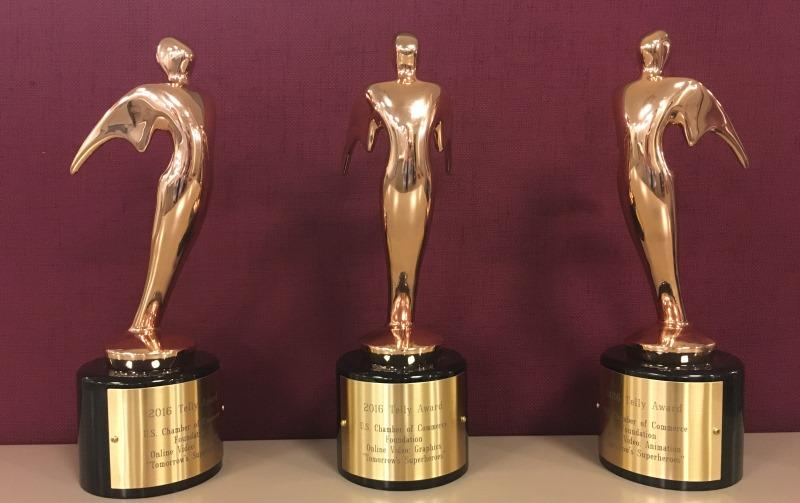The image features three 2016 Telly Awards trophies displayed against a deep velvet red background that casts dramatic shadows onto the table and backdrop. Each trophy features a gold, abstract humanoid figure with no discernible limbs, facing forward while projecting their chest and stretching their arms backward. The trophies are identically designed, with their bases in black and plaques in gold. They read "2016 Telly Award," "U.S. Chamber of Commerce Foundation," "Online Video Graphics," and "Superheroes." The central trophy faces the camera directly, while the trophies on the left and right are angled towards the middle trophy. All three trophies are placed on a light-colored table, creating a striking contrast with the rich, maroon background.